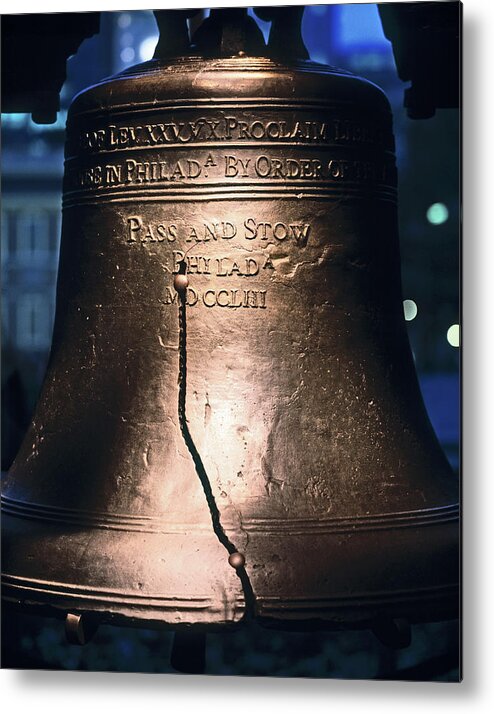The image prominently displays the iconic Liberty Bell, distinguished by its notable crack. The bell is suspended and crafted from bronze with a golden-brown hue. Engraved at the top are embossed words, including "Pass and Stow," with a partially obscured Latin inscription, likely referring to its creation and significance to Philadelphia. The bell features a large, visible crack famously associated with its history. In the background, an out-of-focus sketch of the White House Capitol building, lit in a bluish hue, is set against a black backdrop. Teal dots, resembling lights, and shadowy edges envelop the scene, enhancing the bell's central illumination.